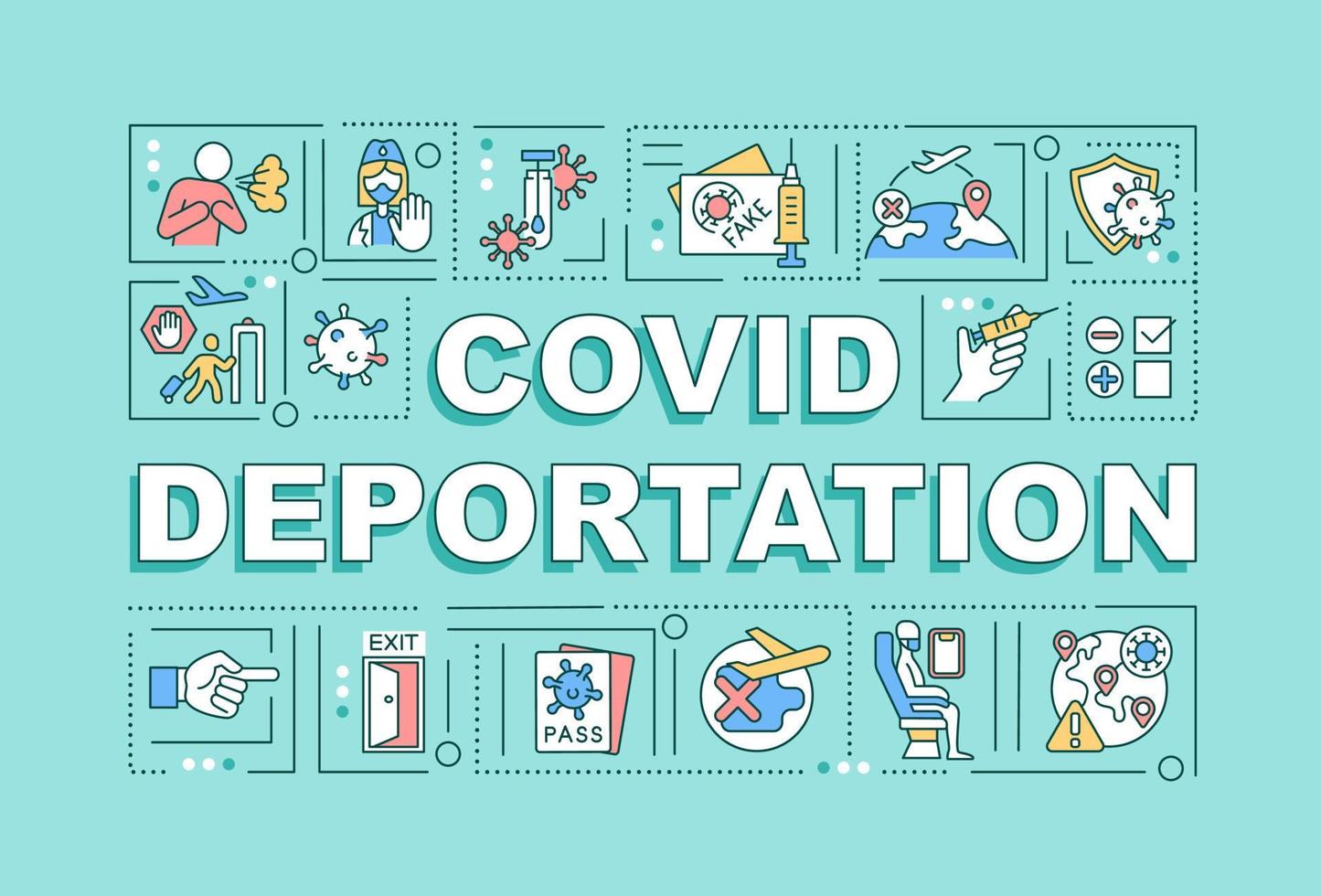This horizontal rectangular image features a mint green background and prominently displays the text "COVID DEPORTATION" in large, all-capital white block letters with a dark outline. Surrounding the central text are 16 smaller squares, each containing different cartoon images. These images include a person coughing, another person wearing a mask with their hand extended, an outline of a syringe, a document reading "FAKE," and an individual sitting in a doctor's chair. Additionally, there are images of an airport metal detector, a door with an exit sign, a hand pointing, an airplane, and a person seated on the airplane. The diverse collection of images, which float around the central text, appears to represent themes of health measures, travel, and possibly deportation related to COVID-19.